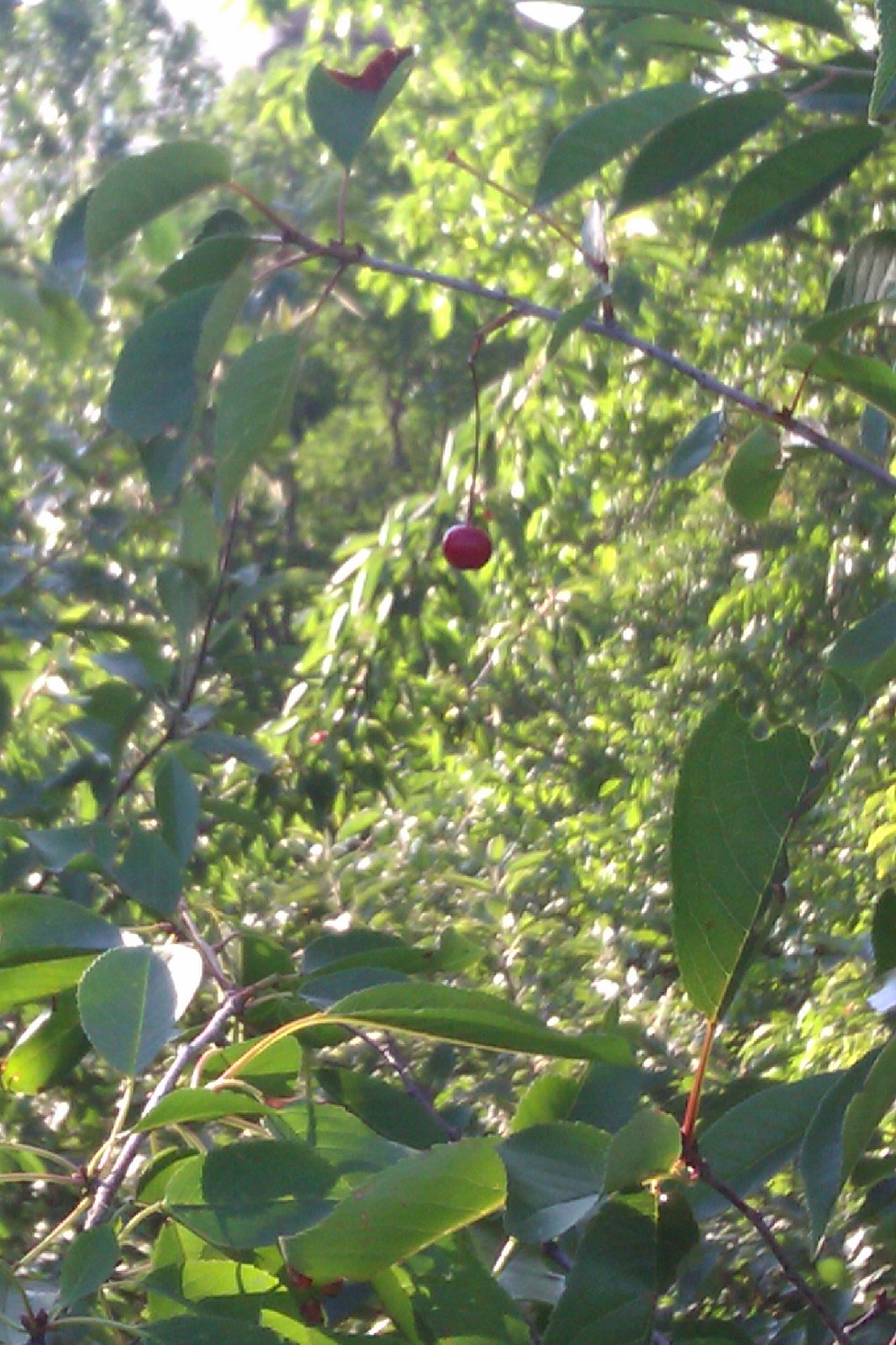In this close-up photograph taken in a lush, dense forest, the focal point is a singular, cherry-like red berry hanging from a thin, brownish-orange twig. The berry, small and circular, dangles prominently in the center of the image. Surrounding it, the scene is teeming with broad, rounded green leaves, some of which have visible insect bites. The thick foliage, composed of scrubby yet non-desert-like trees, fills the picture, with the green leaves reflecting the sunlight that filters through the canopy. The background, slightly blurred to emphasize the berry, shows a mix of green leaves and the muted grayish tones of plant stalks. Though the sunny day is evident from the light reflections and the glimmers of sunlight making their way through the leaves, the exact position of the sun remains indistinguishable.